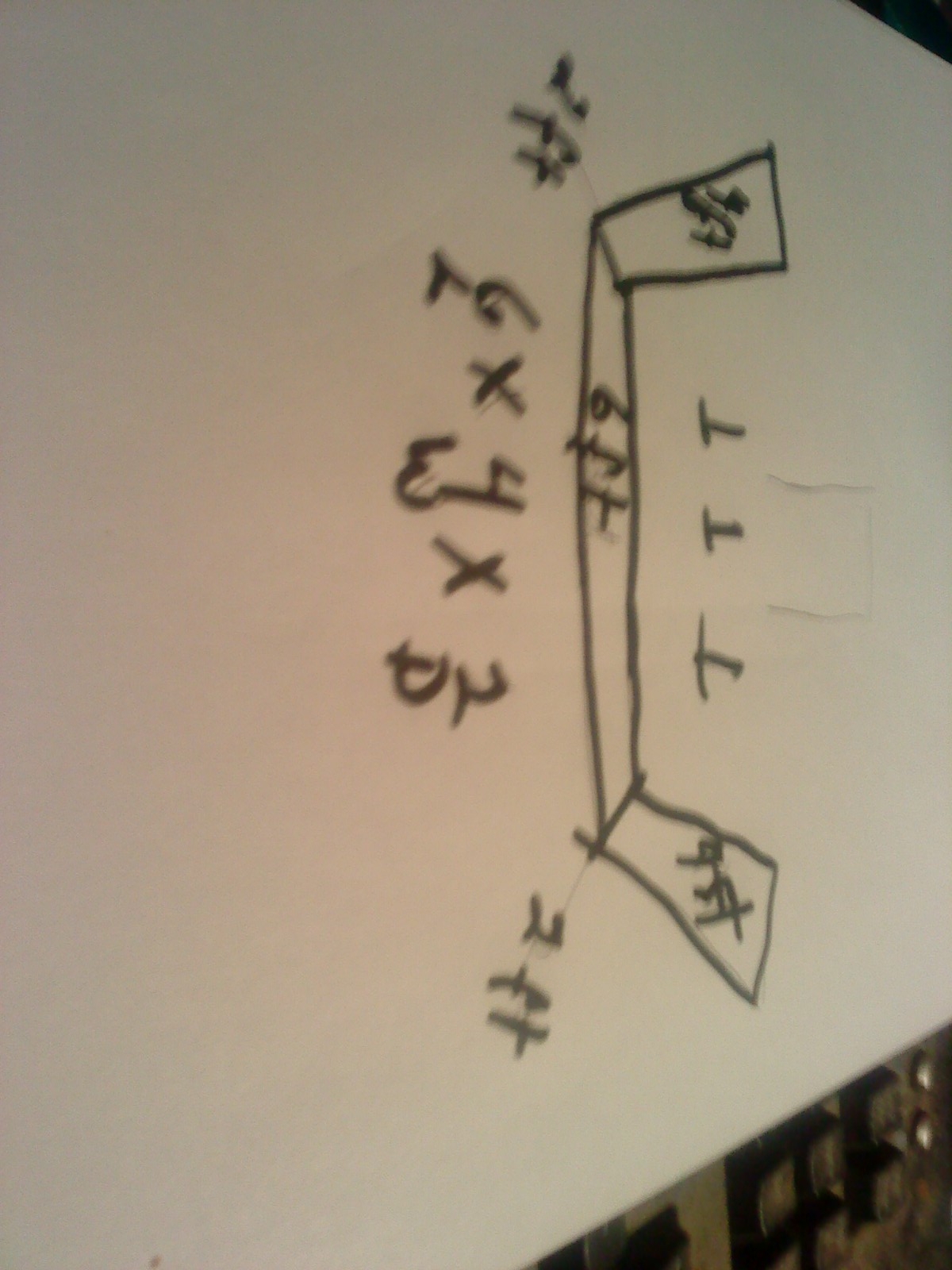The blurry, out-of-focus photograph depicts a piece of horizontal white paper featuring hand-drawn dimensions, numbers, and lines. Oriented sideways, the numbers on the paper have their tops facing the right and their bottoms facing the left, suggesting the camera was held sideways when the photo was taken. The paper, tapering off into the background towards the right, occupies the left side of the frame, with a small black triangle visible in the upper right corner and a black computer keyboard in the lower right corner.

The drawn image on the paper includes a prominent U-shaped figure marked as six feet wide. The right branch of this U-shape is labeled nine feet, while the label on the left branch is illegible. Above this figure, towards the right, are three upside-down T marks accompanied by additional numbers. Below these adjustments, it reads "2 feet", followed by dimensional specifications written as "6' L", "4' W", and "2' D". The overall drawing has been annotated to specify a depth of two feet.

Executed in black pen or marker, the lines of the drawing are uneven and wobbly. The photograph’s lack of focus and clarity further obscures the details, making the entire composition appear blurry.